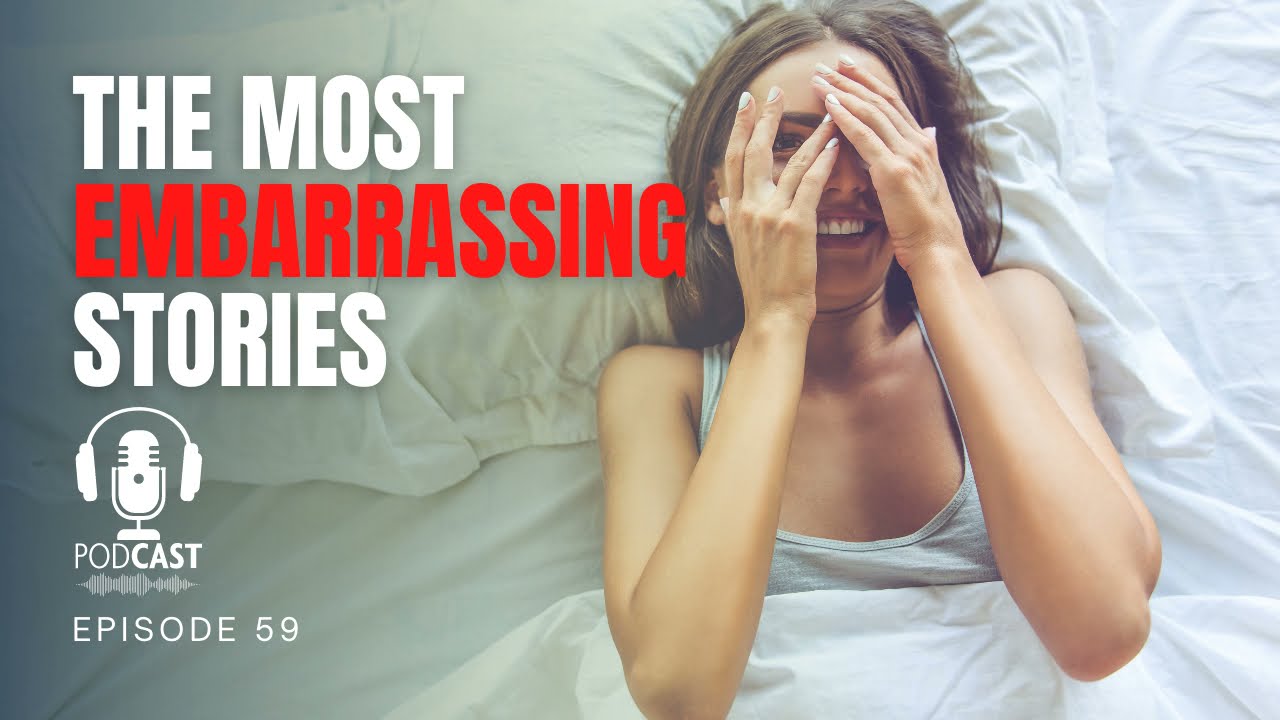This thumbnail image for Podcast Episode 59 prominently features a joyful woman with long brown hair, lying on a bed with white sheets and a white pillow. Viewed from above, she has her hands partially covering her face, revealing her wide smile and the gleam in one eye. Clad in a gray tank top with the bed sheets pulled up to her chest, the scene captures the light source coming from the right, illuminating the white sheets on that side while casting a shadow on the left.

In the upper left corner of the image, bold text announces "THE MOST EMBARRASSING STORIES," with "MOST" and "STORIES" in white capital letters and "EMBARRASSING" strikingly in red. Below this, there is a logo featuring a microphone wrapped with headphones, accompanied by the white text "PODCAST EPISODE 59." The overall layout and the vibrant elements suggest a light-hearted podcast session dedicated to sharing and laughing over the most mortifying stories.